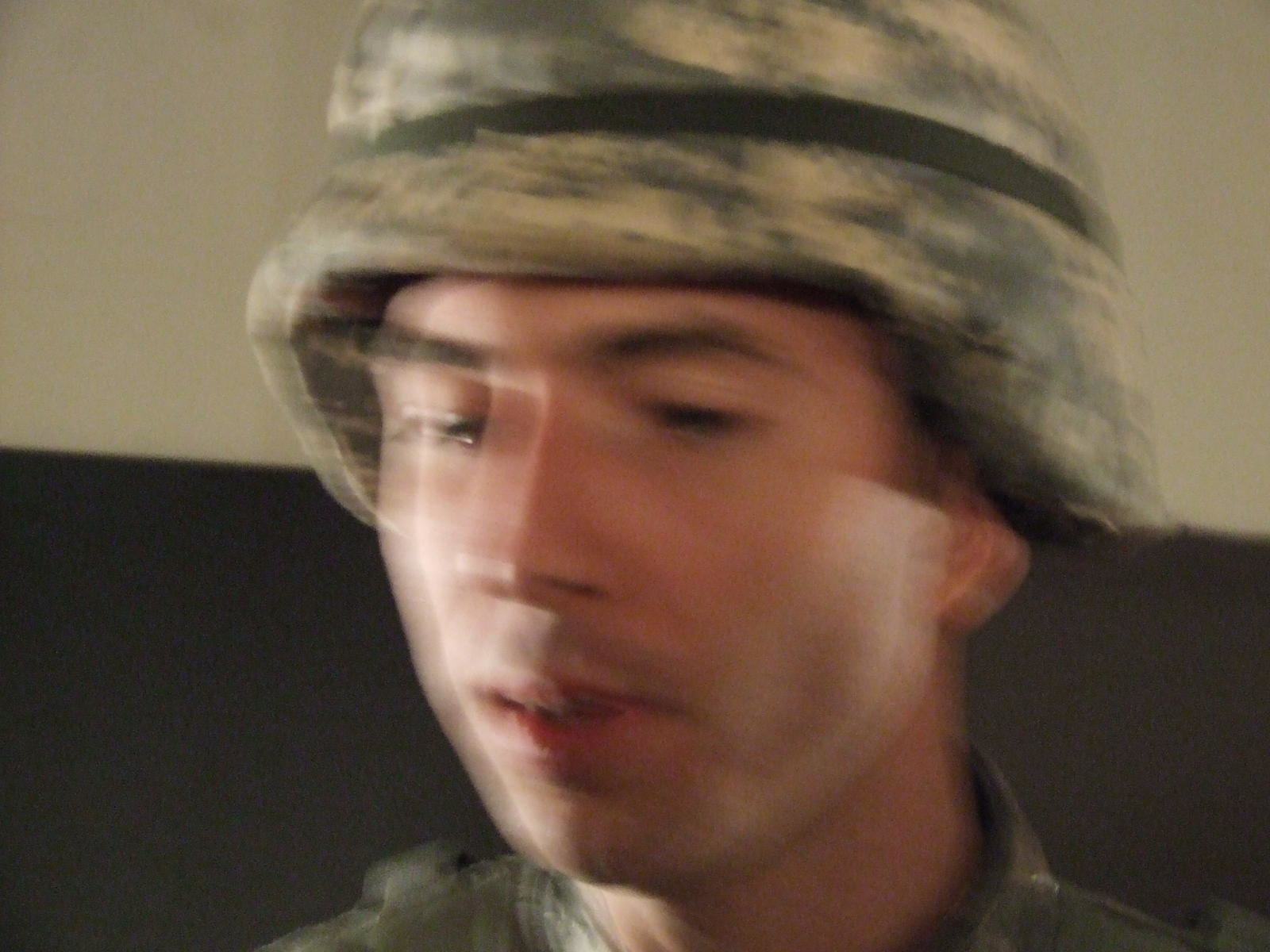The image features a close-up shot, focusing on a man's face from just below his neck to about two-thirds of his head. The man is wearing a rounded hat, reminiscent of a helmet, decorated with the distinctive camouflage pattern commonly associated with the US Army. A black band encircles the hat. The man's gaze is directed downward, and he has relatively brown skin and a thin nose. The photograph is blurred, likely due to camera movement during the shot.